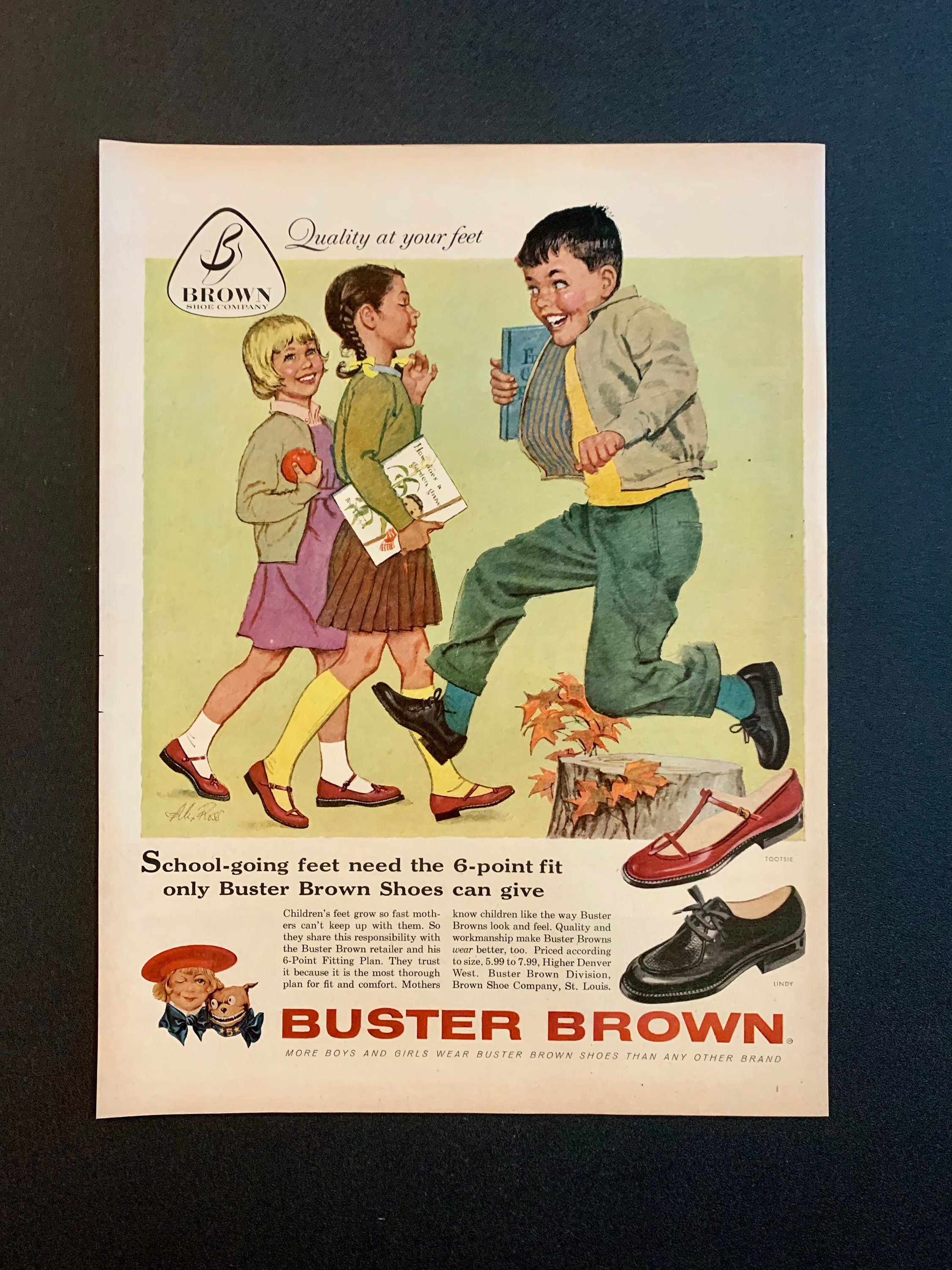A nostalgic magazine advertisement from the 60s or 70s for Buster Brown Shoes, featuring a detailed Norman Rockwell-style illustration of three joyful school children mounted on a black background. At the top, the text reads "Quality at your feet" with the phrase "Brown Shoe Company" mentioned. The advertisement shows a boy in a beige jacket, green pants, and black dress shoes holding a blue book, energetically skipping next to two girls who are also adorned in Buster Brown shoes. The blonde girl, dressed in a purple dress and green jacket, holds an apple, while the girl with ponytails wears a brown skirt, green jacket, and yellow socks. Both girls wear red Mary Jane shoes, enhancing the vibrant scene. Below the illustration, the text states, "School-going feet need the six-point fit only Buster Brown shoes can give," accompanied by two paragraphs of persuasive content and a prominent red "Buster Brown" inscription at the bottom. The advertisement is further enriched by the playful Buster Brown logo, depicting the boy in a red beret and his wide-eyed dog, emphasizing the brand's slogan: "More boys and girls wear Buster Brown shoes than any other brand." To the right are images of two pairs of shoes: one brown and one black, highlighting the available options for young feet.